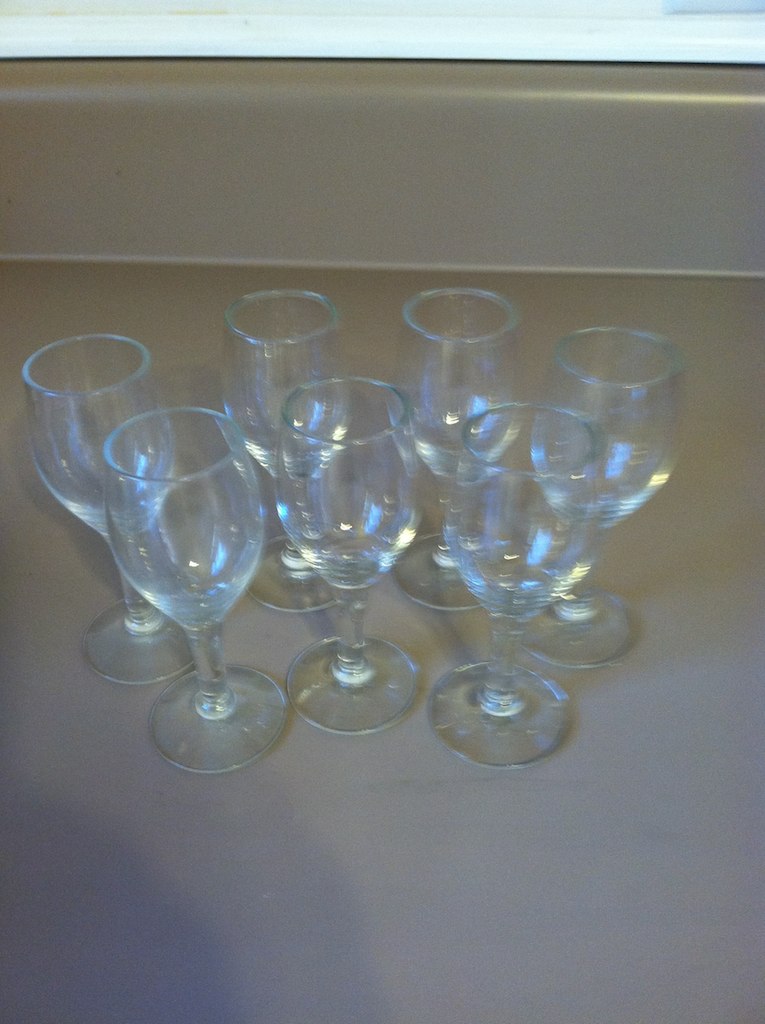The photograph captures a top-down view of seven clear wine glasses arranged in a semi-circle, with four in the back and three in the front, on a beige surface that appears to be a countertop. The setting resembles a kitchen, possibly one found in a nursing home, judging by its plain, tan appearance. The background consists of a matching beige wall or backsplash, with some white trim at the top. The image is somewhat blurry, suggesting it was taken in motion or out of focus, and a shadow is visible in the bottom left corner. The scene is devoid of any additional items or text, giving it a rather minimalistic and straightforward appearance, much like a photo one might see in a classified ad for selling the glasses.